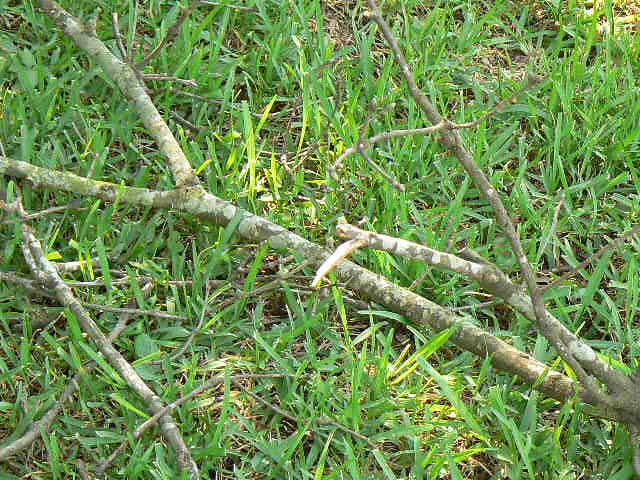This daytime photograph captures a grassy outdoor area with a variety of detailed elements. The grass is mostly green, but there are patches where it appears yellow, possibly due to sunlight shining down on those spots. Scattered across the grass, particularly in the left bottom corner, are several smaller twigs. A larger, multi-branched tree limb, devoid of leaves and colored in shades of brown, green, and a little bit of gray, stretches diagonally from the bottom right corner to the top left. This prominent branch splits into three arms, with the middle one being notably shorter and cut off. Amongst the grass, which is thick and long, some bare patches of dirt are visible, enhancing the natural, somewhat untended look of the scene.